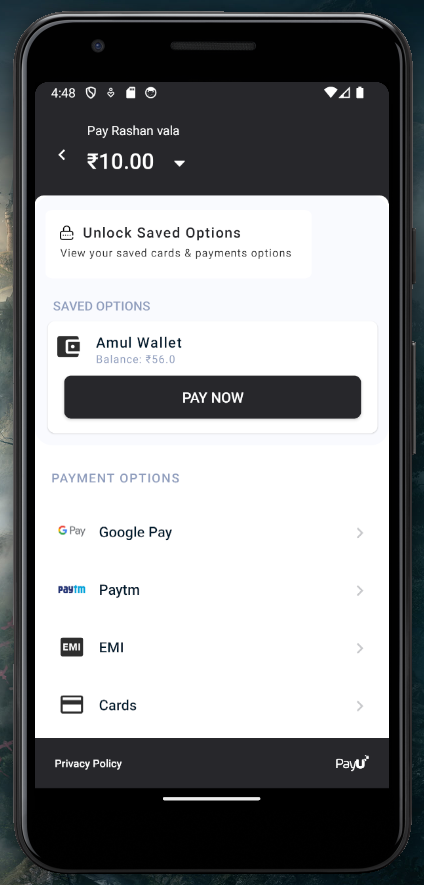A detailed screenshot depicting a smartphone in profile view. The top-left corner features the current time, four standard notification icons, while the top-right corner shows Wi-Fi connectivity and battery life percentage. Below the notification bar, the screen displays a payment interface with a prompt to "pay Rishan Vala" an amount of 10.00 in the local currency, denoted by a less-than sign (<) pointing to the left.

Midway down the screen, a white rectangular pop-up box presents the saved payment options. Within this box, viewers can see various saved cards and payment methods including:

1. **Amul Wallet** with a balance of 56.
2. A black "Pay Now" button for executing transactions.

Further payment options listed under the pop-up box include:
1. GPay (Google Pay),
2. Paytm,
3. EMI cards.

This highly detailed interface illustrates the comprehensive payment methods available for the transaction, ensuring a secure and efficient digital payment experience.